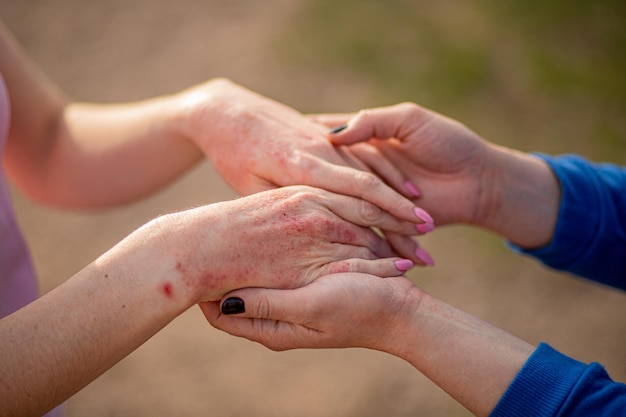In this landscape-oriented photo, two people are holding hands, creating an intimate and detailed image. The background is out of focus, displaying patches of green and tan, with a dominant peach hue. The person on the right is dressed in a long-sleeved blue shirt, the sleeves slightly rolled up, and has black nail polish. Their hands, positioned beneath the other's, exhibit a firm yet gentle grasp. On the left, the individual wears a purple shirt, revealing arms up to mid-forearm. Their hands, positioned on top, are notable for pink nail polish and a visible skin condition characterized by red, bumpy, and irritated patches, suggesting a rash or some skin ailment. This vivid detail enhances the viewer's perception of a tender moment amidst shared vulnerabilities.